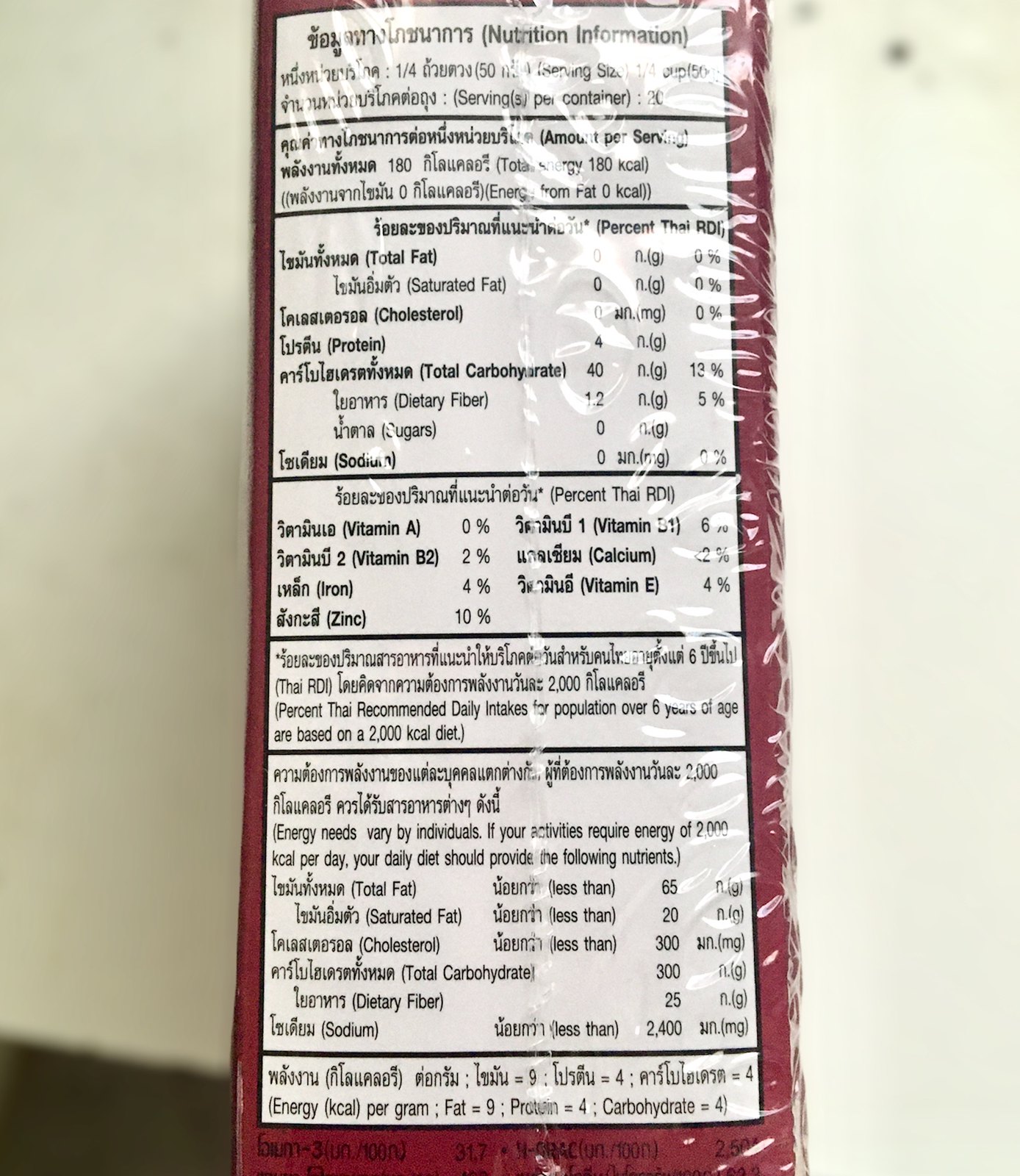This detailed image showcases a nutritional panel on the rear side of an elongated, rectangular box. The entire back surface is dominated by the nutritional information label, which appears to be printed in a foreign language, possibly Turkish. Encapsulating the box is a clear plastic film, with visible wrinkles particularly prominent along the right side and extending slightly to the bottom. The box is positioned on a white countertop, which, though somewhat blurred, emphasizes the contrast with the packaging. Additional black text in a foreign script is evident below the nutritional panel, adding to the box's informative layout.